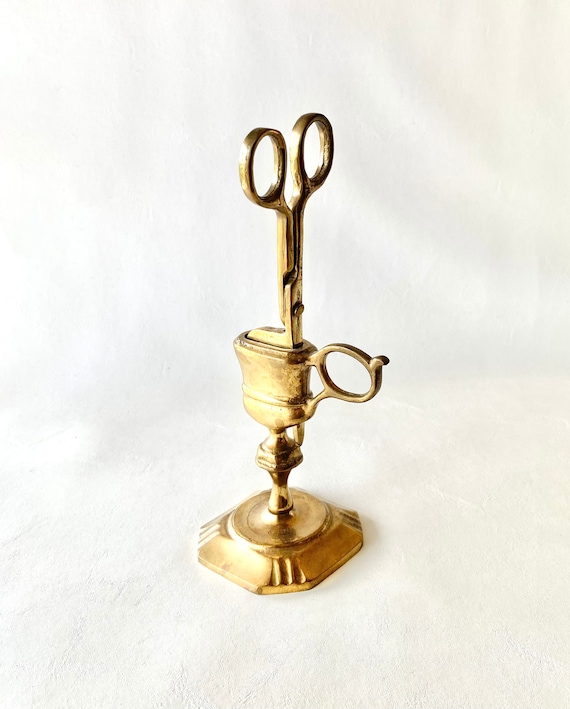The image showcases a color photograph in portrait orientation, featuring a brass stand designed to hold a pair of scissors. Set against a white background, the stand is the central focus of the image, presenting a tall and narrow structure positioned on what appears to be a flat, white surface. The base of the stand is a squared shape with its corners slightly beveled, creating the appearance of a hexagonal or octagonal figure. Extending upward from the base, the stand has a circular handle on its right side, ensuring a secure grip. At the pinnacle of the stand, a pair of brass scissors is inverted, with the blades inserted into a dedicated opening at the top. The scissors are positioned diagonally, with their finger holes tilted towards the left at the top and the cutting ends pointed downward. The overall style of the image emphasizes photographic realism, capturing the intricate details and gold luster of the brass stand and scissors against an abstract, cream, and gray patterned backdrop.